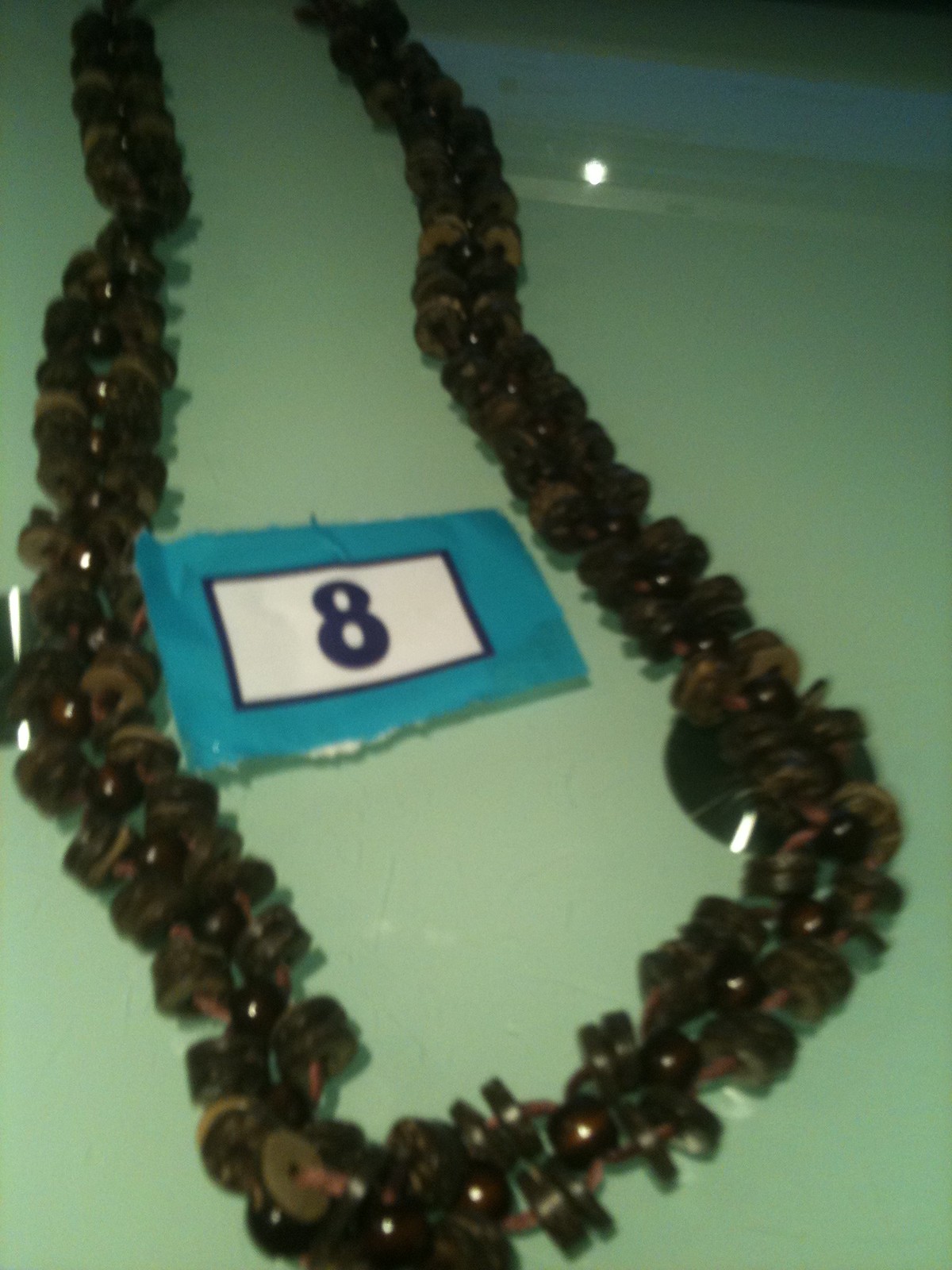The image depicts a somewhat blurry photograph of a large necklace, likely displayed in a museum or exhibit. The necklace is intricately made up of brown, circular beads that resemble buttons, as well as interspersed wooden round beads woven together in two parallel chains. Its overall design suggests a form similar to a Hawaiian lei, but instead of flowers, it features these beads. The beads are strung on brown or bronze-colored cording. The necklace is placed on a light green, shiny surface, possibly a plastic tray, which reflects light and nearby objects. In the center of the necklace, there is a blue, square placard with a ripped appearance. Inside this blue placard, a white box prominently displays the number eight in dark blue.